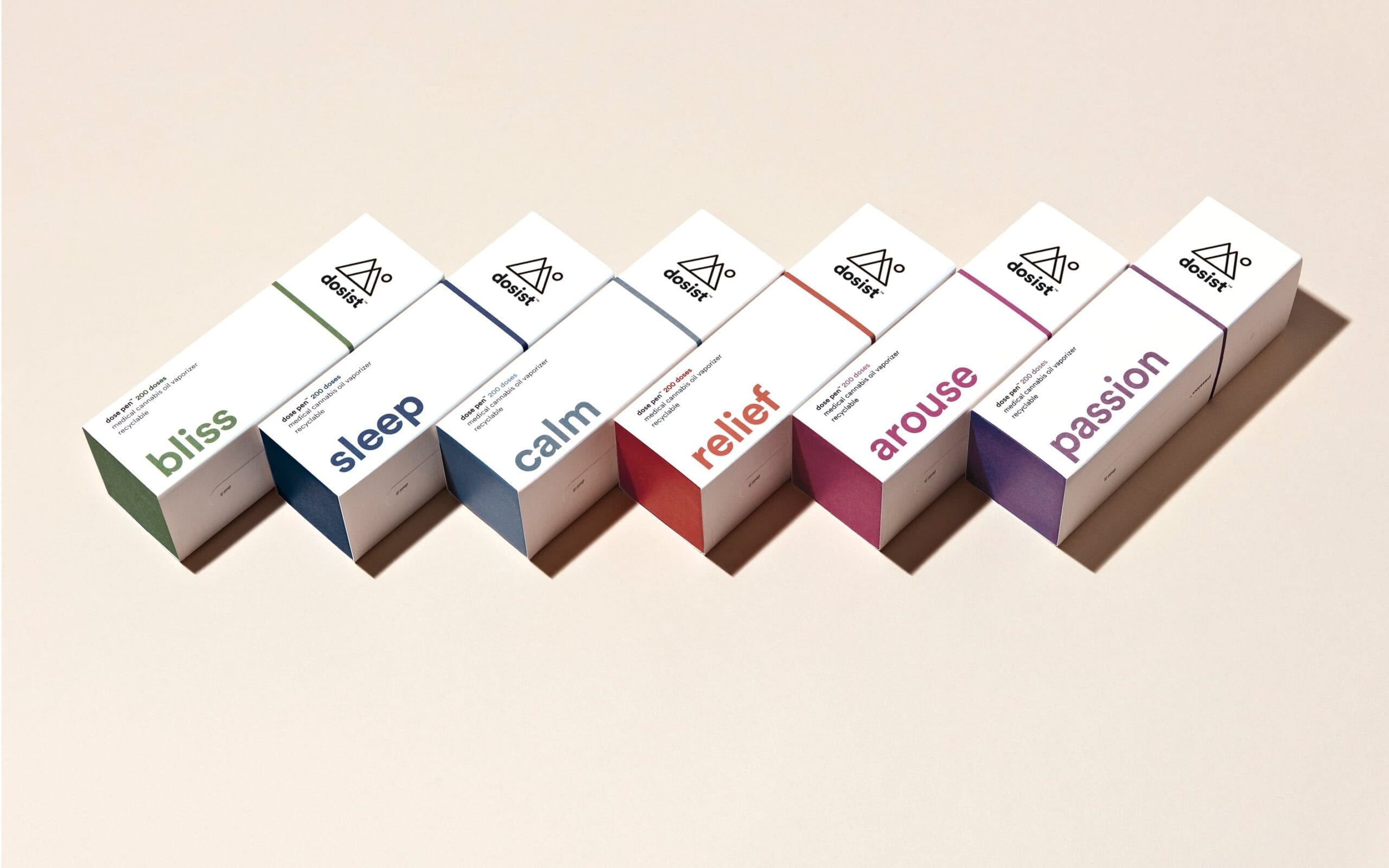This photograph features six sleek, rectangular boxes from the company dosist, each distinguished by a different color and label indicative of its intended effect. From left to right, the labels and colors are: bliss in green, sleep in navy blue, calm in light blue, relief in red, arouse in magenta, and passion in purple. Each box is predominantly white with black text displaying the brand name "dosist" at the top, accompanied by an icon consisting of two overlapping triangles, forming an M shape with a small circle, resembling a moon, nearby. The consistent and stylish design suggests these could be products like essential oils or incense, each tailored to evoke specific feelings or states of mind.